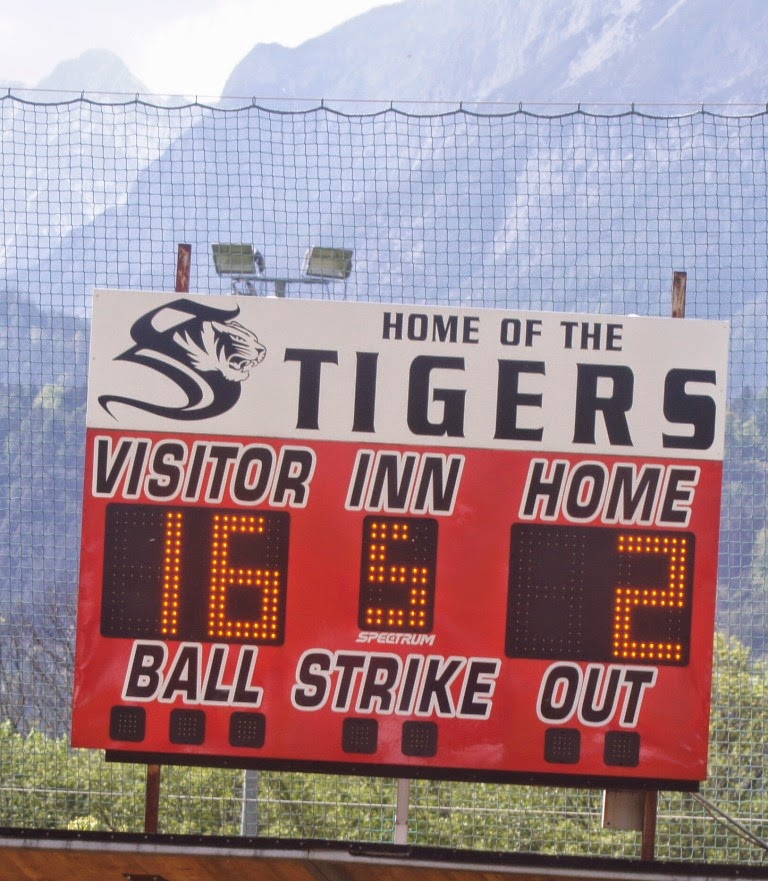The photograph captures an outdoor scoreboard at a minor league or school sports stadium. Dominating the image, the scoreboard is prominently white on top and red on the lower section, with the text "Home of the Tigers" and a logo featuring an 'S' and a tiger head. Below this, the scoreboard displays details such as "Visitor," "INN" (Inning), and "Home," with the current score showing the visitors leading 16 to 2 in the fifth inning. The sections for "Ball," "Strike," and "Out" are indicated but not illuminated. In the background, there is netting behind the scoreboard, trees, and green foliage, with pale, purplish-blue tinted mountains or high hills stretching across the top of the image. The scene suggests a serene outdoor sports field situated close to scenic mountainous terrain.